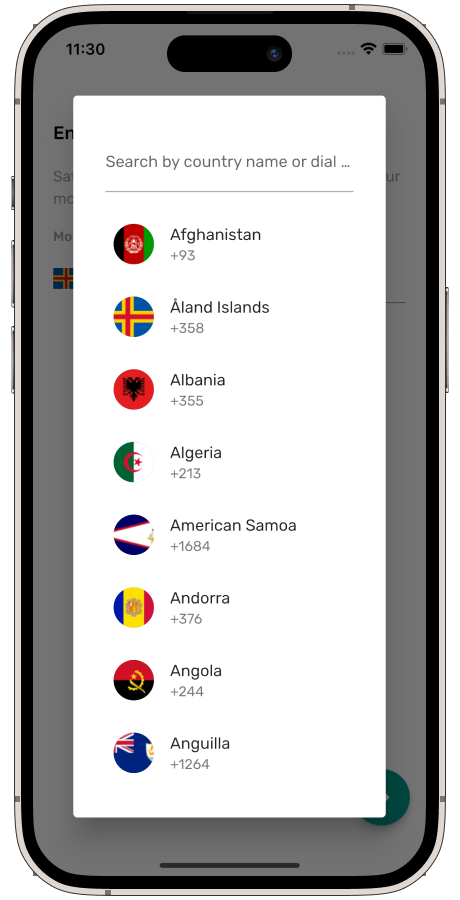The image prominently features a smartphone displaying a pop-up menu with various country flags and their corresponding international dialing codes. The pop-up allows users to "search by country name or dial." Here are the visible details:

- Afghanistan: The popup shows the Afghanistan flag (red, green, and black) with the code "+93".
- Åland Islands: Displaying a flag of blue, red, and yellow, and the code "+358".
- Albania: Featuring a red and black flag alongside the code "+355".
- Algeria: Displaying a green, red, and white flag with the code "+213".
- American Samoa: Represented with a black and white flag and the code "+1684".
- Andorra: Showing a flag that is orange, yellow, and red, with the code "+376".
- Angola: The popup displays a flag colored in black, red, and yellow with the code "+244".
- Anguilla: Featuring a flag in red, white, and blue and the code "+1264".

The smartphone in the image indicates that it has a full battery and is connected to Wi-Fi, with the time displayed as 11:30 AM.